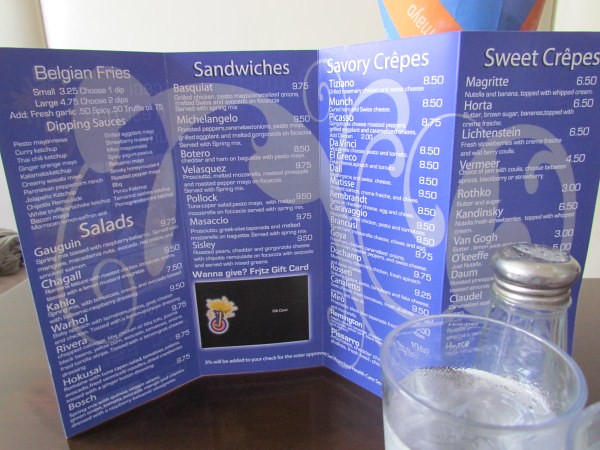In the image, the background features a pristine white wall, creating a clean contrast with the black surface on the ground. Positioned in the bottom right corner is a cup, with a hint of water nearby, suggesting a cool ambiance. Adjacent to the cup sits a salt shaker, distinguished by its silver top and white salt inside. An unfolded menu is visible, presenting an array of culinary offerings.

The top left section of the menu highlights Belgian fries, situated centrally alongside a variety of sandwiches. To the immediate right are savory crêpes, accompanied further right by a selection of sweet crêpes. The leftmost section lists several items including small and large portions, "juice one dip" and "juice two dip," with an additional option to add fresh garlic. 

Further down, the menu features a selection of teas, specifically a "50 spice tea," and a comprehensive list of dipping sauces. These include four standard dipping sauces, along with specialty dips such as tex, salad, lemon garlic, chivaro, aglio, warhol, gruyere, carmelado, miso, remington, and pisado. The sweet crêpes section lists unique varieties such as maigrette, harta, wittgenstein, vermeer, rothko, kadinsky, van Gogh, O'Keefe, Dom, and Claudel, showcasing an extensive range and creative naming conventions.